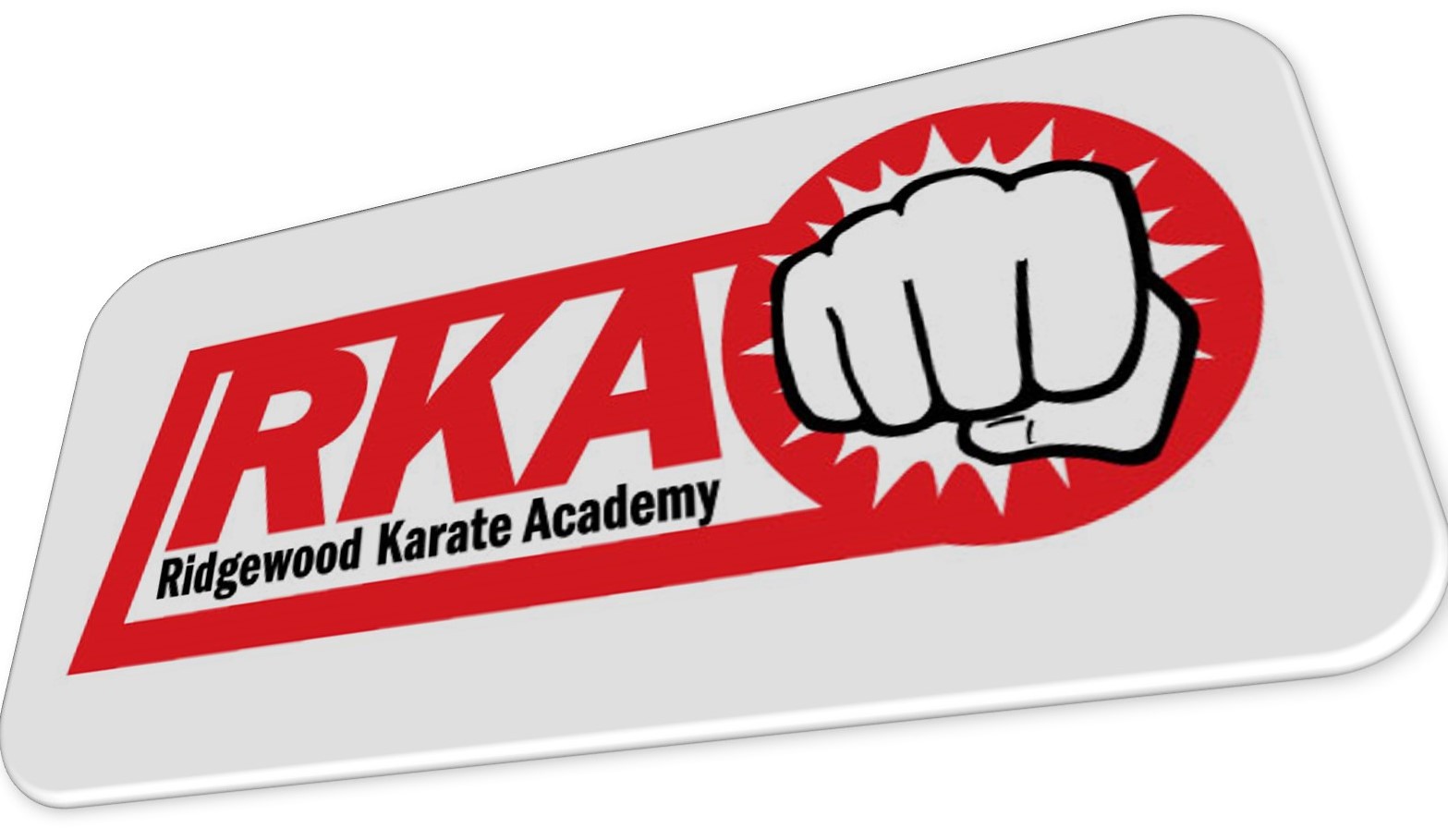This image features a detailed 3D rendering of a rectangular name tag with rounded edges, depicted against a pure white background, emphasizing its freestanding presence. The name tag itself is off-white, enhancing its three-dimensional appearance with noticeable shadows and curves along the edges. At the center of this tag is a vivid red logo that encapsulates the brand identity.

The logo comprises a medium-red rectangle on the left intersecting with a red circle on the right. Inside the circle, there's an outlined black fist with a jagged, white explosion effect surrounding it, giving a dynamic impression of impact. Within the red rectangle, 'RKA' is written in bold red text, while 'Ridgewood Karate Academy' appears below it in black text. This complete logo is precisely centered on the tag, creating a balanced and eye-catching design that clearly represents the Ridgewood Karate Academy.